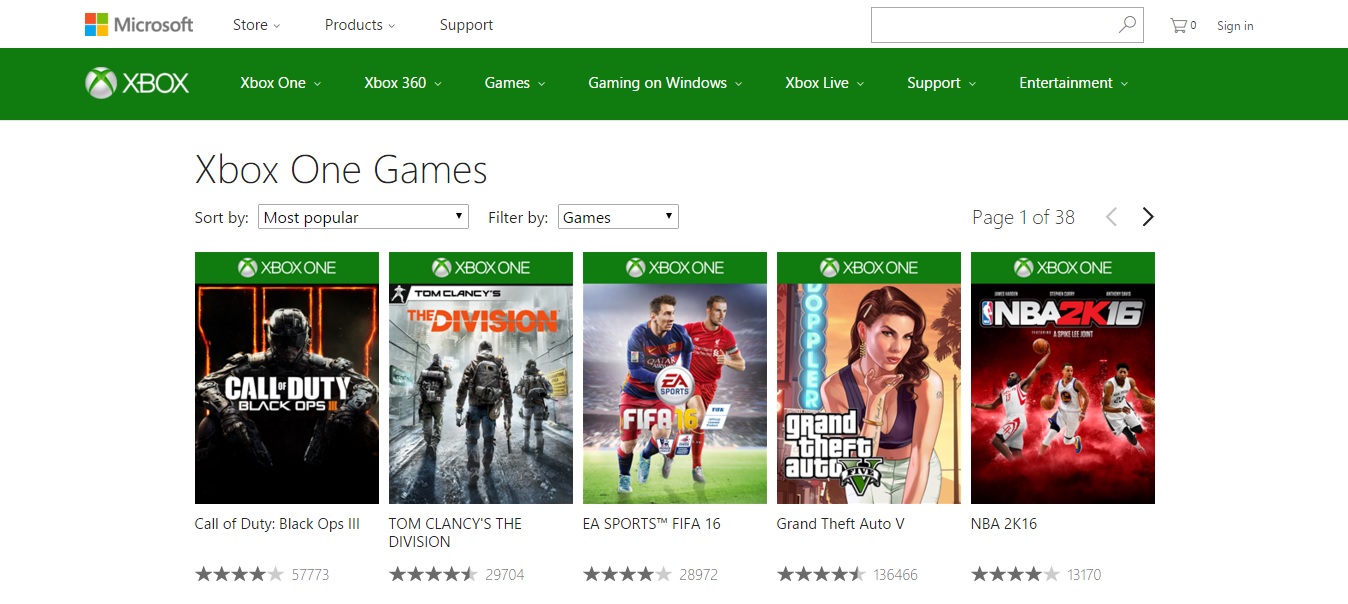In this image set against a pristine white background, the upper left corner features the word "Microsoft" in dark gray text alongside their iconic logo composed of four squares in red, green, blue, and yellow. To the right, a menu includes options such as "Store," "Products," "Support," followed by a search bar, a shopping cart icon, and a sign-in option. 

A vivid green banner spans the width of the image just below this. On the far left of the banner is the word "Xbox" accompanied by a white circle enclosing a green 'X'. The navigation menu on the banner reads "Xbox One" with a pull-down arrow, "Xbox 360" with a pull-down arrow, "Games," "Gaming on Windows," "Xbox Live," "Support," and "Entertainment."

Below this banner, in gray text against the white backdrop, is the heading "Xbox One Games." Displayed from left to right are the following games: "Xbox One Call of Duty: Black Ops," which boasts a rating of four out of five stars based on 57,773 reviews. Next is "Xbox One The Division," subtitled "Tom Clancy's The Division" in gray text below it.